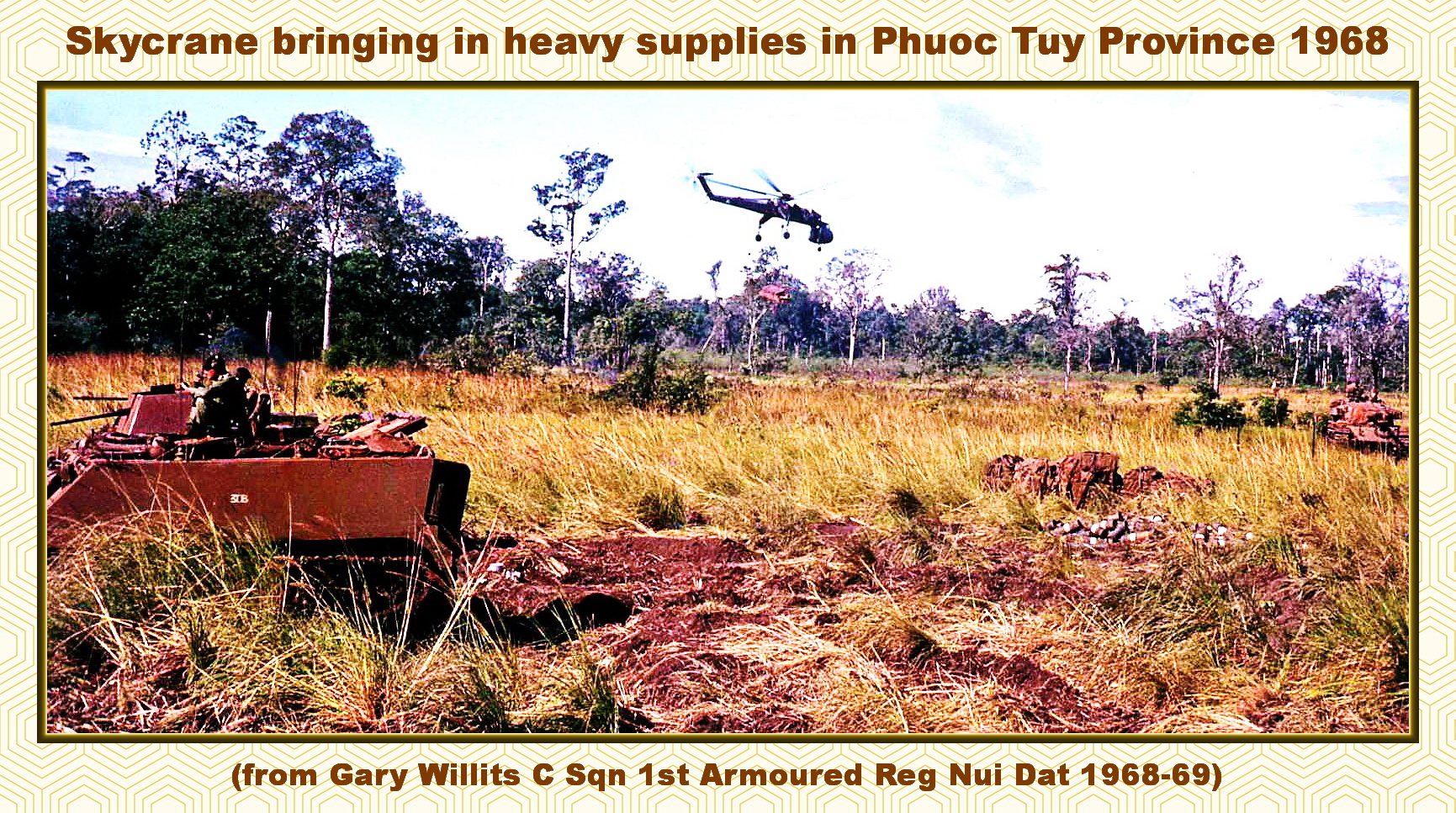The vintage wartime photograph, framed within a textured tan border featuring a hexagonal pattern, captures a scene from Phuoc Thai province in 1968. At the top, there's a header in brown text that reads, "Skycrane bringing in heavy supplies in Phuoc Thai province 1968," while the bottom of the image is captioned, "From Gary Willits C.SQN 1st Armoured Reg, Newadar 1968-1969."

The image itself prominently displays a cloudy daytime sky over a grassy field, dotted with dirt piles or holes. In the background, a dense forest lines the horizon. In the foreground, several tanks and armored vehicles are seen, including a square armored vehicle with a turret and a person atop it on the left side of the frame. Another tank is visible on the right. High above, a helicopter, identified as a Skycrane, soars through the sky. Notably, this specialized helicopter has a distinct cockpit at the front, dangling wheels, a thin central body, and top-mounted propellers, indicating its role in transporting heavy supplies. The photograph is a poignant snapshot of military operations during the Vietnam War.